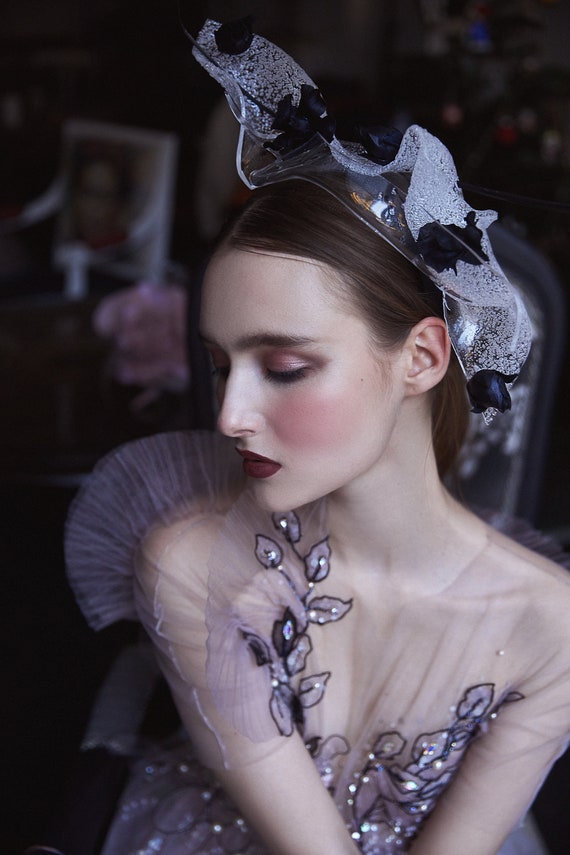The image features a striking young woman, likely in her late 20s or early 30s, dressed in a delicate, frilly lavender dress designed with theatrical flair. The sheer, almost see-through fabric, adorned with purple, silver, and black floral and leaf patterns, wraps gracefully around her body. The dress is accentuated with sequins and a purplish plant motif on transparent lace. Her head is adorned with an unusual clear plastic headpiece, wrapped in white and blue fabric connected to plexiglass, giving the impression of a fairy-like or ballerina ensemble. Her heavy makeup includes vividly red cheeks, red lipstick, and red eyeshadow, enhancing her striking beauty. She dominates the image, exuding a sense of vanity and poise, with a blurry background that does not detract from her presence.